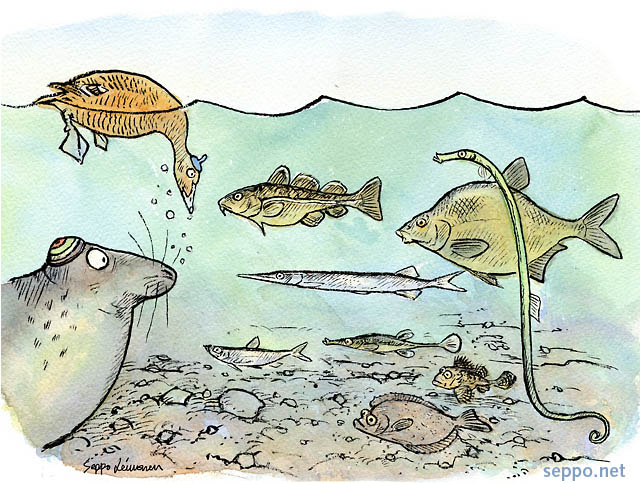This vibrant color illustration by Cepo.net depicts a whimsical underwater scene filled with various sea creatures. The cross-section view reveals a light blue sky without clouds and a blue-green ocean with visible ripples on the surface. Near the water’s surface on the left, an orange duck wearing a blue hat has its head submerged, seemingly interacting with a greenish fish that resembles a sea bass. Below the sea bass, a long, silver swordfish swims gracefully. On the bottom left, a gray sea lion or seal wearing a colorful striped hat gazes at the other sea creatures. Interspersed throughout the scene are smaller fish in hues of green, silver, yellow, and brown. Towards the right side, an amusingly wide and fat fish, colored green and yellow, floats next to a very thin fish resembling a seahorse. The ocean floor is dotted with small rocks and pebbles, completing this enchanting cartoon depiction of underwater life.